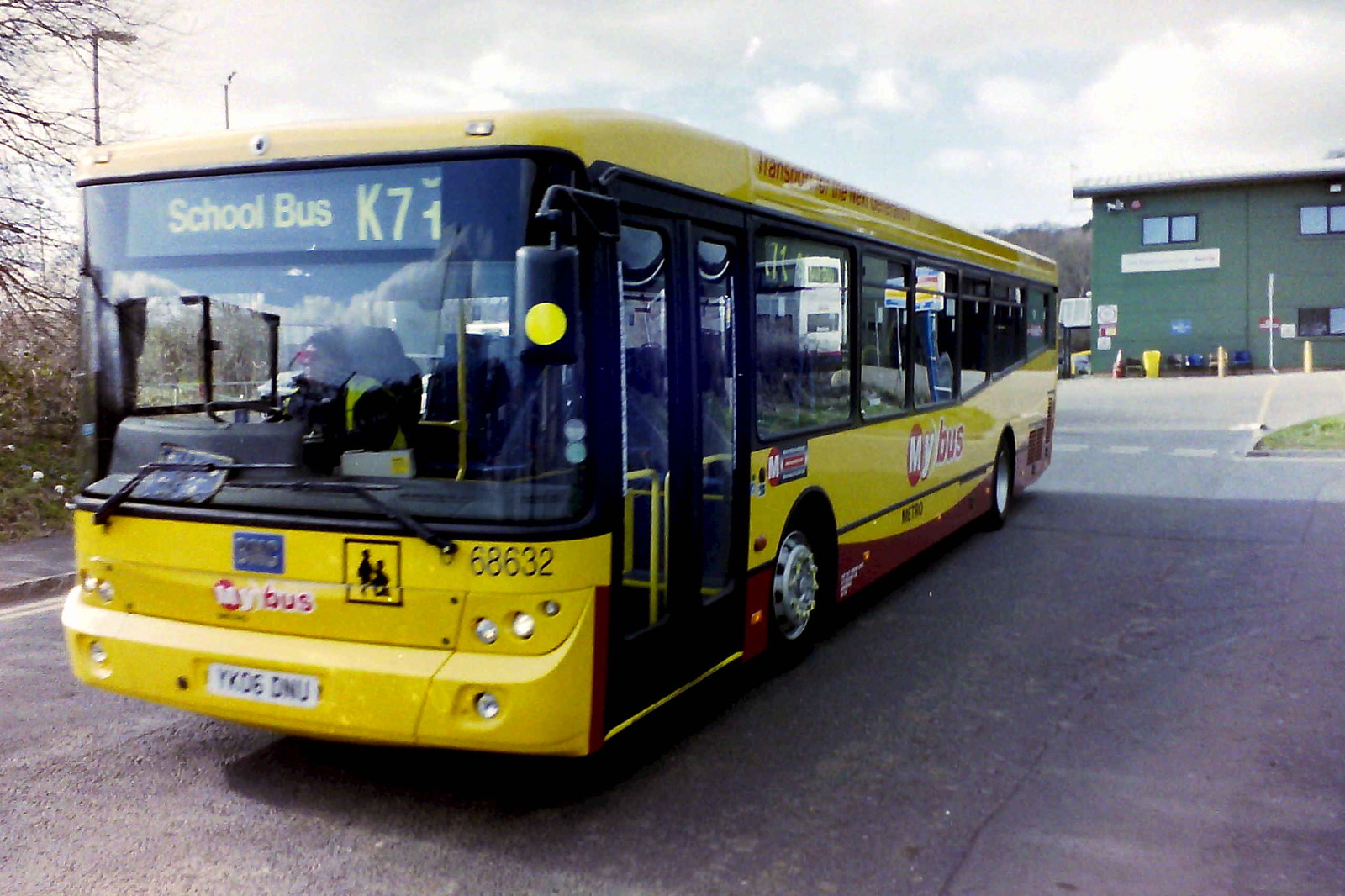This image features a bright yellow school bus, prominently marked with the designation "School Bus K71" above the windshield, and the number "68632" displayed on its body. The bus is parked on a paved road in a city, adjacent to a large green building seen in the background on the right. The bus has red trim at the bottom, and a logo reading "My Bus" on the right side near the entrance. The entrance door, located on the right side of the bus, is open, revealing a bus driver inside who is wearing a hat and a yellow vest. The front of the bus is flat, and the license plate reads YK06D. The background features a somewhat overcast sky with clouds, trees, a sidewalk on the left, and streetlights and poles.